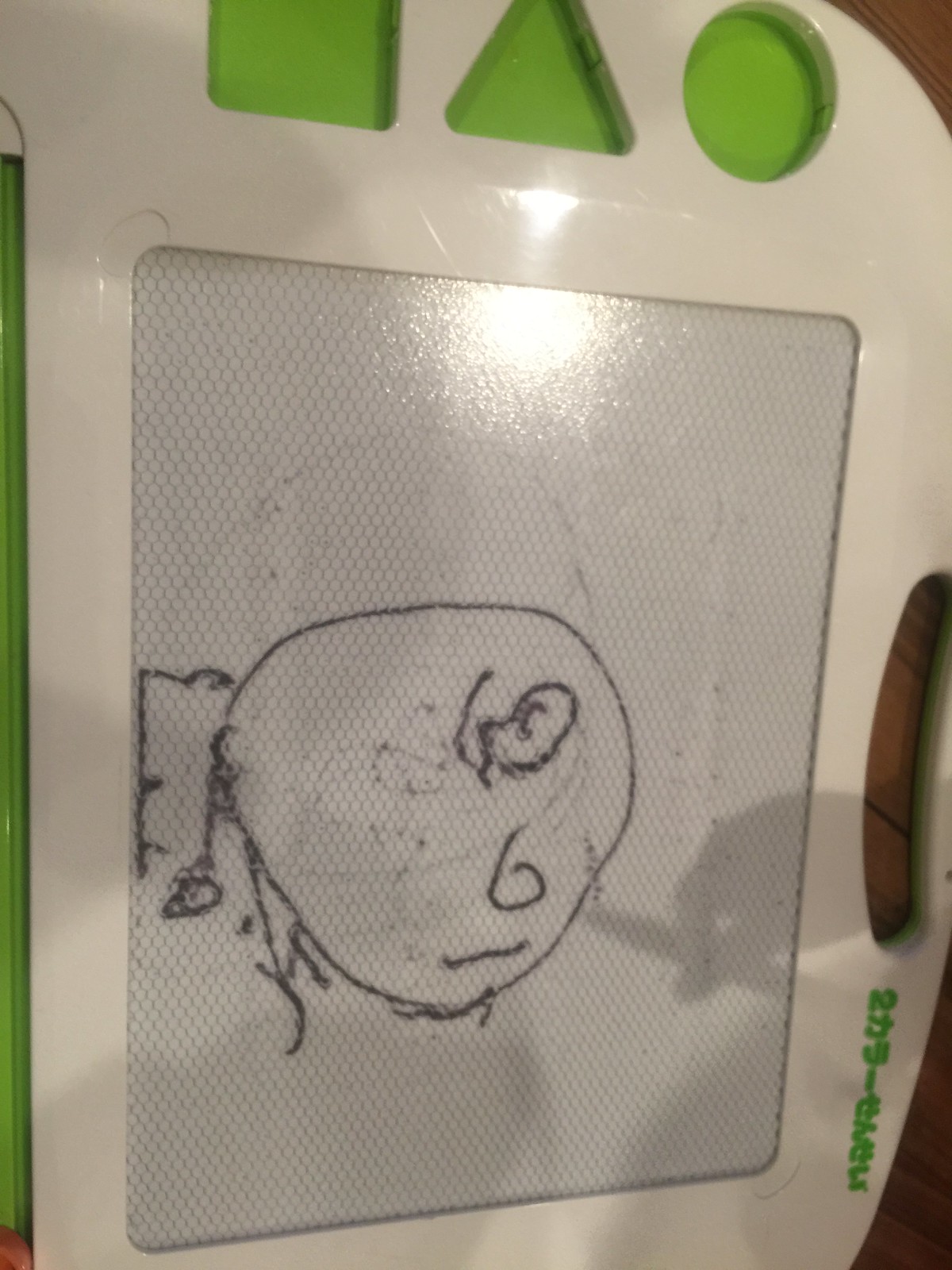This photograph captures a drawing similar to an Etch-a-Sketch, a popular children's toy known for its magnetic-based display. The device features a white plastic frame with a handle at the top, and is set on what appears to be a brown wooden table. The top of the toy has Chinese or Japanese characters, indicating potential international origins or inspiration. On the left side of the frame, there are three geometric cutouts: a green square, green triangle, and green circle.

The drawing itself appears to be the work of a child, indicated by the imperfect large circle that represents a face. Inside the circle are two squiggly shapes for eyes and a horizontal line underneath, likely meant to depict a mouth. Extending from the circle are long black lines symbolizing arms. A shadow of a person's finger holding a writing utensil is also visible, emphasizing the interactive nature of this toy. The back of the drawing pad features a pattern of small white diamond shapes, adding a textural contrast to the overall design.